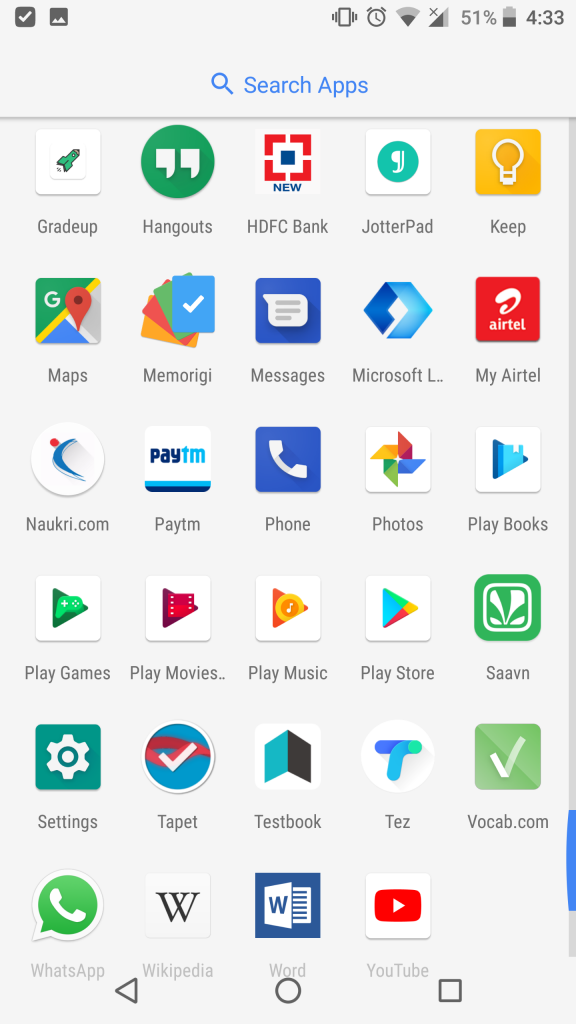In this image, we see a detailed screenshot of a smartphone interface against a light gray background. 

In the upper left corner, a white check mark is visible inside a black box. Next to it is an icon for "Photos." Moving to the right, we observe a series of status icons: an alarm clock, a Wi-Fi symbol, a battery indicator showing 51%, and the time displayed as 4:33.

Below these status icons, there is a search bar with blue text that reads "Search apps" accompanied by a magnifying glass icon in the center. 

The screen is organized into rows of app icons:
1. First row (left to right): "Grader," "Hangouts," "HDFC Bank," "JotterPad," and "Keep" (which is represented by a yellow square with a white light bulb).
2. Second row (left to right): "Google Maps," "Memory," "Messages," "Microsoft," and "My Airtel."
3. Third row (left to right): "Naukri.com," "Paytm," "Phone," "Photos," and "Play Books."

Below this, separated by a line, are more app icons listed from left to right: "Play Games," "Play Movies," "Play Music," and "Play Store."